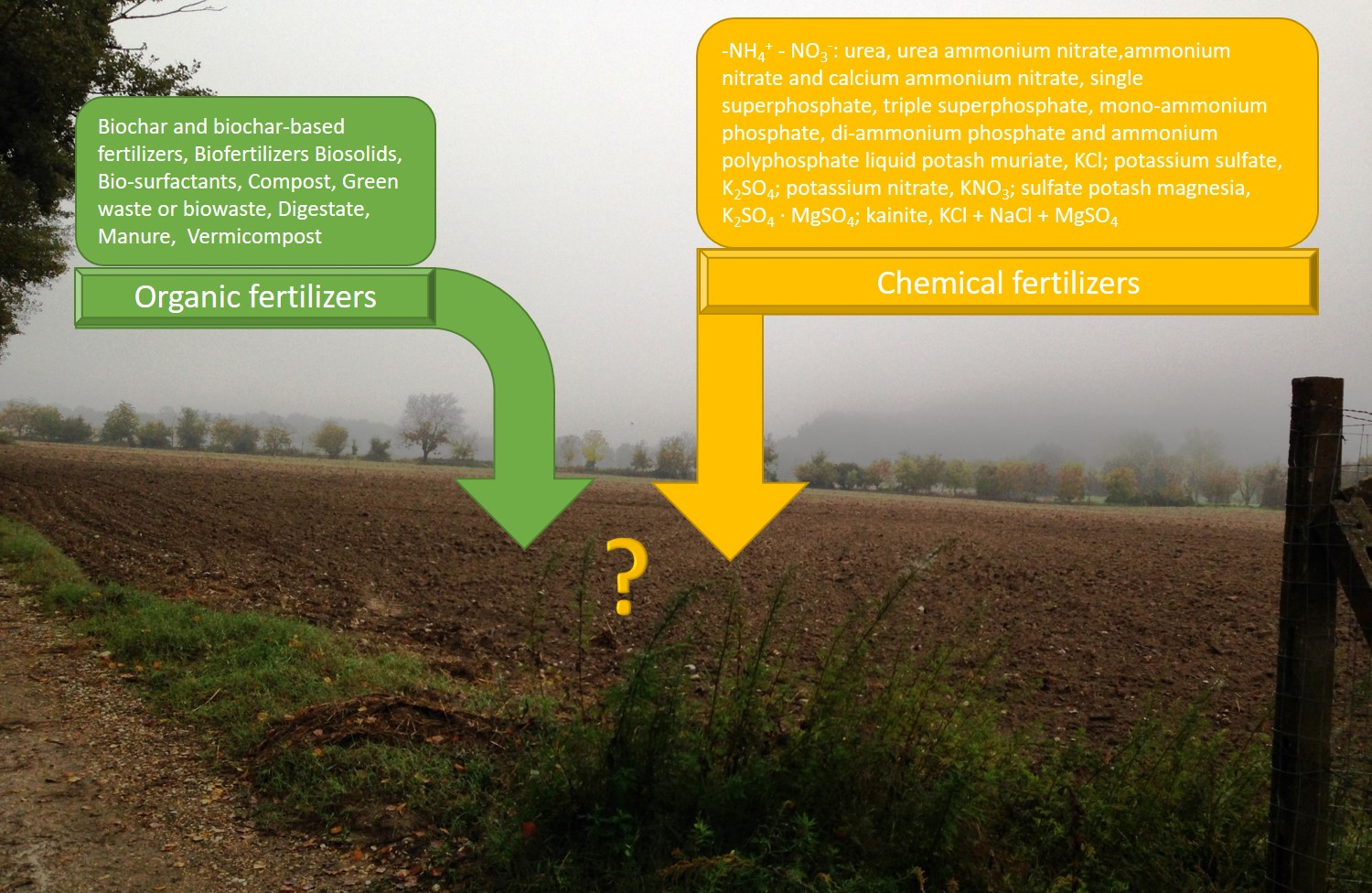The image depicts a rectangular, outdoor field scene, photographed from a wide-angle perspective under a gray, stormy sky suggesting an overcast and possibly midday setting. The field is predominantly dark brown and appears to be tilled, with some patches of green grass and foliage along its edges. Trees, including many evergreens, line the background, framing the scene with a sense of seasonal transition, possibly late fall. 

Central to the image is a striking yellow question mark, placed between two detailed, computer-generated signs. The sign on the left is green with white lettering, listing various organic fertilizers such as biochar, biochar-based fertilizers, biofertilizers, biosolids, biosurfactants, compost, green waste, bio-waste, digestate, manure, vermicompost, and organic fertilizers. An arrow from this green sign points downward towards the field, indicating these materials' application to the land.

To the right, a yellow sign with black lettering enumerates various chemical fertilizers, including compounds like NH4+, NO3-, urea, ammonium nitrate, calcium ammonium nitrate, single superphosphate, triple superphosphate, monoammonium phosphate, diammonium phosphate, ammonium polyphosphate, liquid potash, KCl, potassium sulfate (K2SO4), potassium nitrate (KNO3), sulfate potash magnesia (K2SO4·MgSO4), kainite, KCl+NaCl, and MgSO4. This yellow sign also features a downward-pointing arrow indicating these chemicals' application to the same field.

Additional visual details include a round fence on the field's right side and a small trail with a tall tree on the left, adding layers of depth and context to this illustrative comparison of organic versus chemical fertilizers.